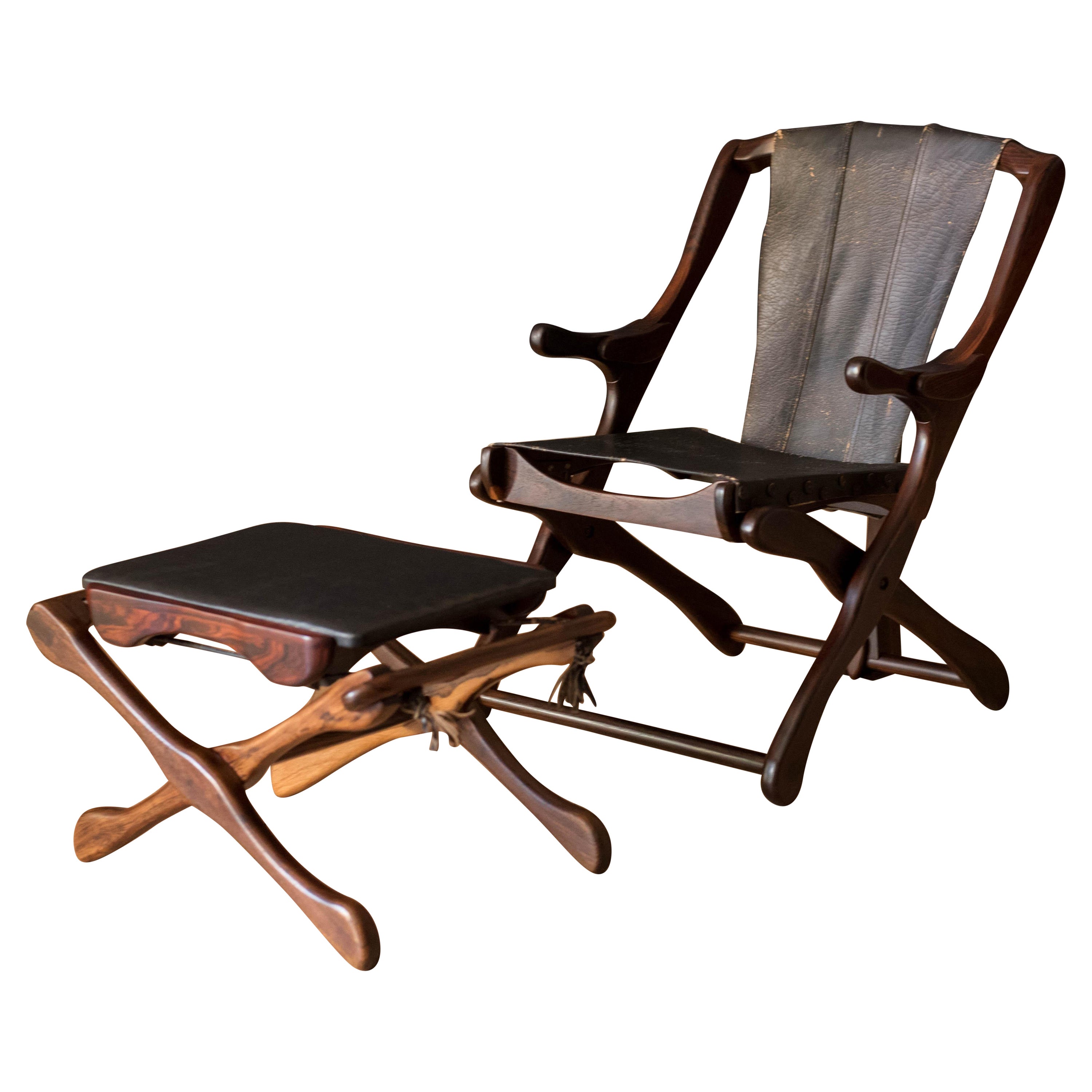The image depicts an antique wooden chair accompanied by a wooden stool that doubles as a small table. The chair exhibits a classic, old-style design, though it does not appear rusted or tarnished. The wooden frame of the chair surrounds a mesh seat area, giving it a distinctive combination of materials. Draped over the middle section of the chair is a cloth or scarf, adding an element of texture. Notably, the chair lacks a backrest, which raises questions about whether it is broken or follows an original design that omits this feature. The stool in front serves a dual function as both a footrest and a small tray-like table, further emphasizing the antique aesthetic.